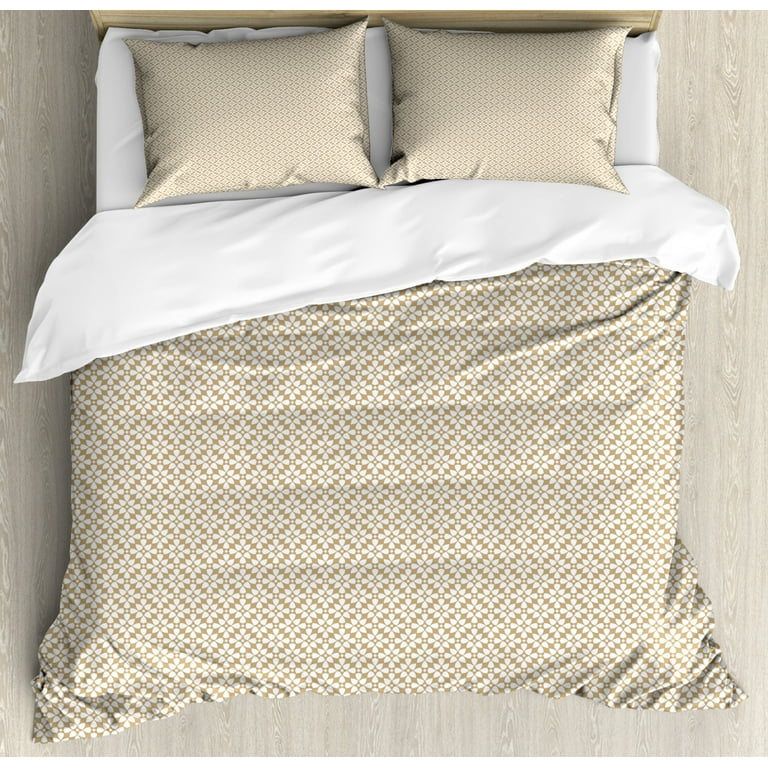This image is an overhead view of a meticulously arranged full-sized bed. The bedspread, a golden white comforter adorned with intricate diamond and square patterns, is slightly pulled back to reveal two pillows at the head of the bed. The pillows, matching the comforter's design with their light golden and light brown hues, feature the same repeated geometric motifs. Beneath the comforter, light sheets peek through, ensuring an invitingly layered aesthetic. The headboard, subtly visible, is constructed of light brown wood, adding a rustic touch to the setup. The floor around the bed, visible along the sides and at the foot, is composed of light brown wood with gray undertones, complementing the overall cozy and warm atmosphere of the bedroom.